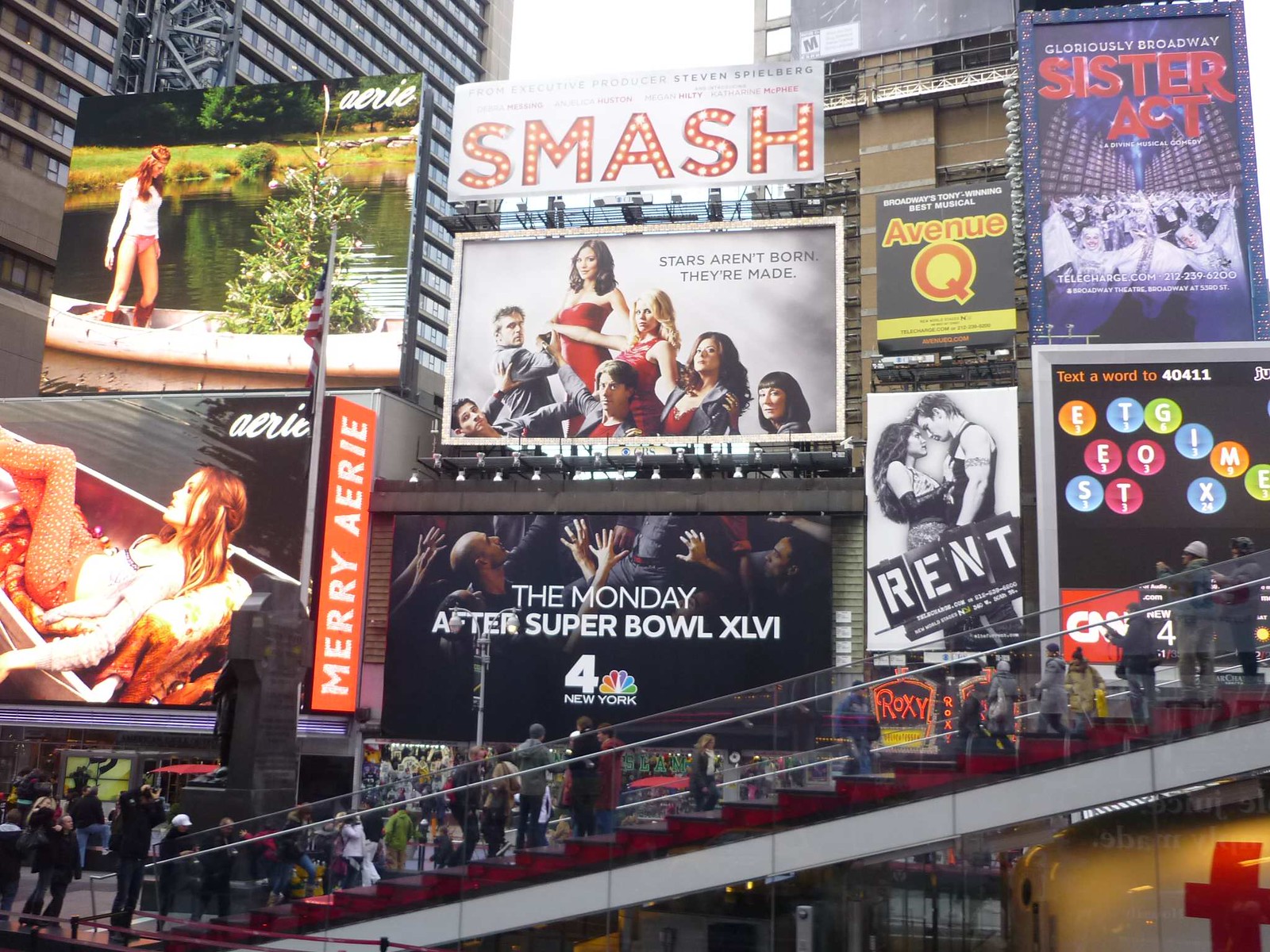This vibrant, outdoor, daytime color photograph captures the bustling atmosphere at a prominent Broadway sign billboard viewing area, located in front of the TKTS booth, identifiable by the visible "T" in the lower corner. The image, taken from street level, showcases a large array of billboards affixed to a building with tall skyscrapers in the background. 

At the forefront, there is a diagonal barrier railing leading to a set of red-painted bleacher steps, filled with people walking up and down, some paused to observe and photograph the vivid advertisements. The billboards are arranged in several rows. Starting from left, there are two Aerie advertisements featuring young women in kayaks, hinting at adventure and outdoor exploration, with the words "Mary Aerie" visible on one.

The central top billboard prominently displays the word "SMASH" in marquee letters, with a tagline below that reads, "STARS AREN'T BORN, THEY'RE MADE." Just beneath, another billboard announces "The Monday After Super Bowl XLVI" with the NBC logo, Channel 4, New York. An assortment of Broadway show advertisements punctuates the right-hand side, including "Avenue Q," "Rent," which depicts a man and woman close together, and "Sister Act," showcasing a group of women in a striking pose.

At the base of the billboards, an escalator filled with people adds to the dynamic energy of the scene, as pedestrians on the sidewalk behind it also look up, drawn to the spectacle of the vibrant advertisements. The overall photographic style is rich in detail and captures the essence of a lively, iconic New York City location.